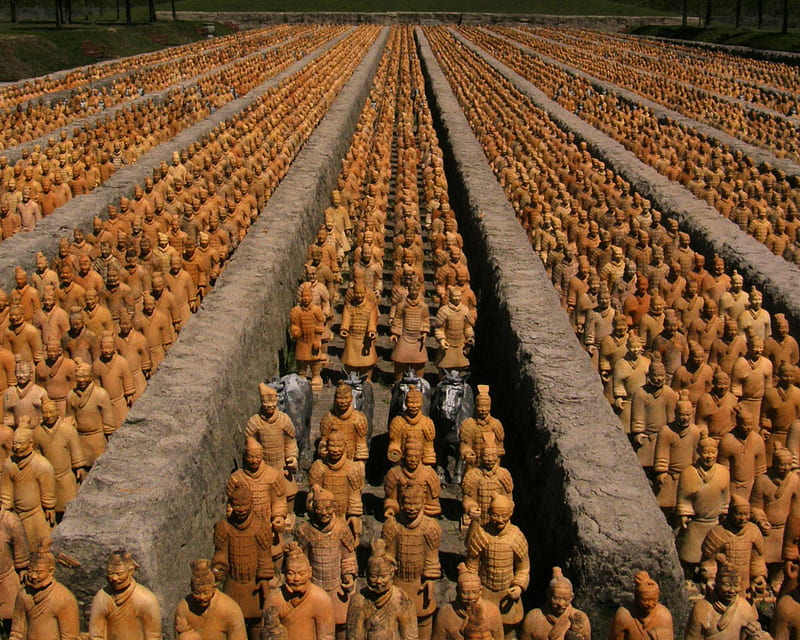This is a detailed landscape-oriented color photograph offering an aerial perspective of the Terracotta Army, located in China. The image captures an impressive assemblage of the Terracotta soldiers, arranged meticulously in rows and columns. Each soldier features distinct Chinese facial characteristics and is adorned in traditional warrior outfits with textured patterns. The soldiers are separated into sections by low concrete walls, creating a sense of order within the expansive room. There are approximately eight visible sections, each containing about four to five rows of these life-sized statues. The scene conveys an overwhelming sense of scale, showcasing hundreds of these intricately carved figures, diminishing in perspective towards the background, highlighting the immense effort and time required to create this monumental archaeological site.